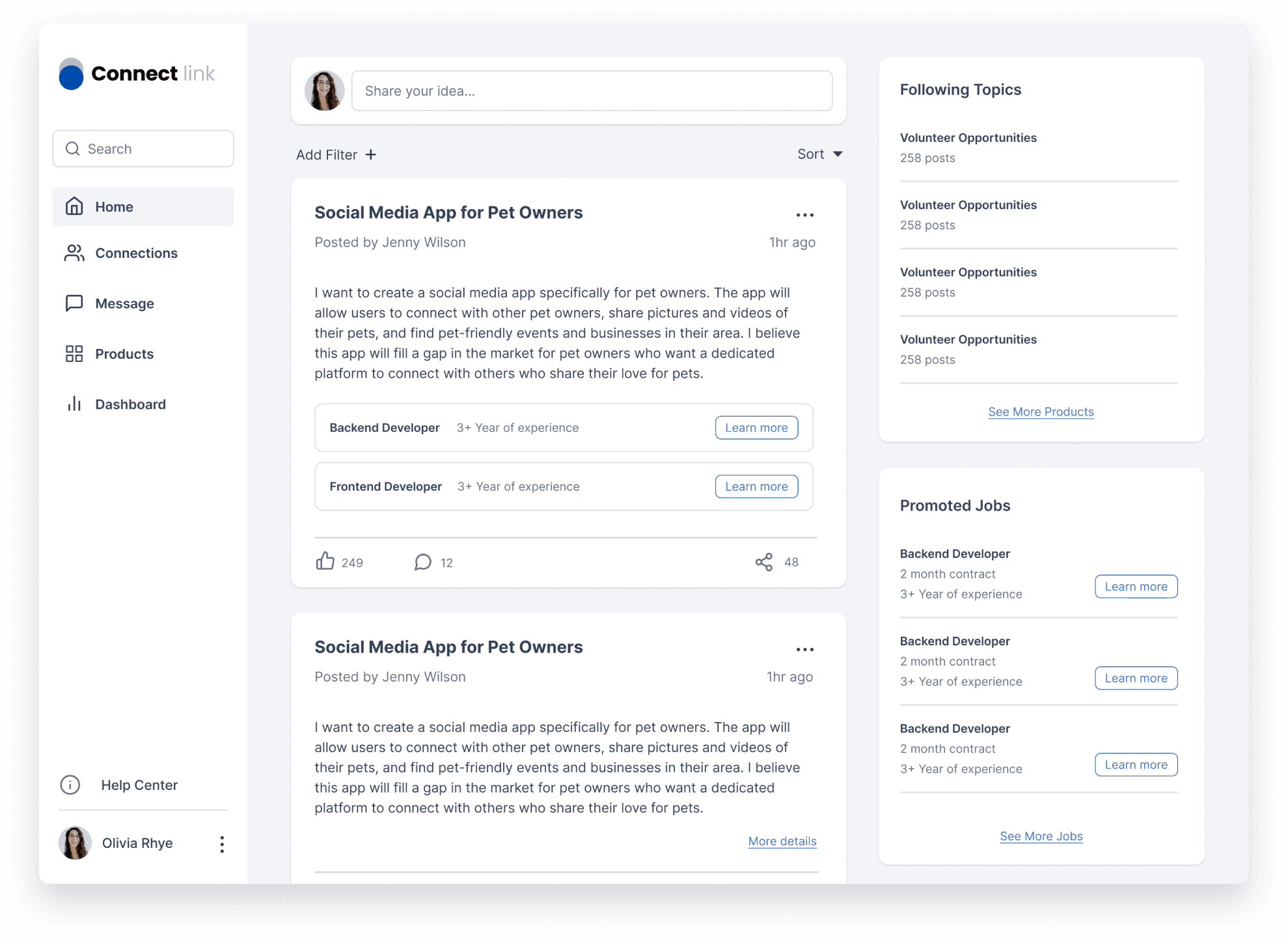This image from ConnectLink's website features a clean and structured layout with a variety of interactive elements. 

On the left side, about two inches inward, is a white background extending from top to bottom. In the top left corner of this area, the brand logo consists of a blue circle followed by the bolded black text "Connect" and the non-bolded text "Link." Below the logo, a search bar runs across from left to right, carrying the placeholder text "search." Underneath the search bar is a home icon followed by the word "home," outlined in gray. Further down this section are labeled buttons: connections, messages, products, and dashboard, each accompanied by their respective icons. 

At the bottom of the left section, there's a photo of a young girl with long hair and glasses, identified as Olivia R-B-Y-A. Directly above her photo, the text "Help Center" is displayed.

The right side of the image has a gray background. In the top left corner of this section, there is a large search bar with the user's profile picture, prompting "share your idea." Below the search bar, a blue-bordered button with black lettering states "add filter," accompanied by a plus sign button labeled "sort."

Underneath these buttons is a large white square containing content related to a social media app for pet owners. The content's header, in bold black text, reads "Social Media App for Pet Owners," with smaller text below noting "posted by Jenny Wilson." This is followed by a five-line paragraph detailing the content. Two tabs span across this section: the first one, labeled "Back End Developer, 3+ years experience," and a "Learn More" tab in white with blue lettering. Below this is another label, "Front End Developer, 3+ years experience," also accompanied by a "Learn More" tab. At the bottom left of the white square are icons: a thumbs-up icon with "249," a talk icon with "12," and a share icon with "48."

To the right of the main content, another white square duplicates the "Social Media App for Pet Owners" post but ends just after the paragraph. This section has a blue header with a white rectangle background titled "Following Topics," listing "Volunteer Opportunities" four times, each with "258 posts" below. Below the fourth entry, a blue text link reads "see more products."

Further down, a white background square is titled "Promoted Jobs" in bold black text, listing three job postings for "Back End Developer, 2 month contract, 3+ years of experience," each with a "Learn More" tab in white with a blue border and lettering. At the bottom of this section, a blue link reads "see more."

This detailed layout ensures users can navigate and interact with various features and information efficiently on ConnectLink's website.